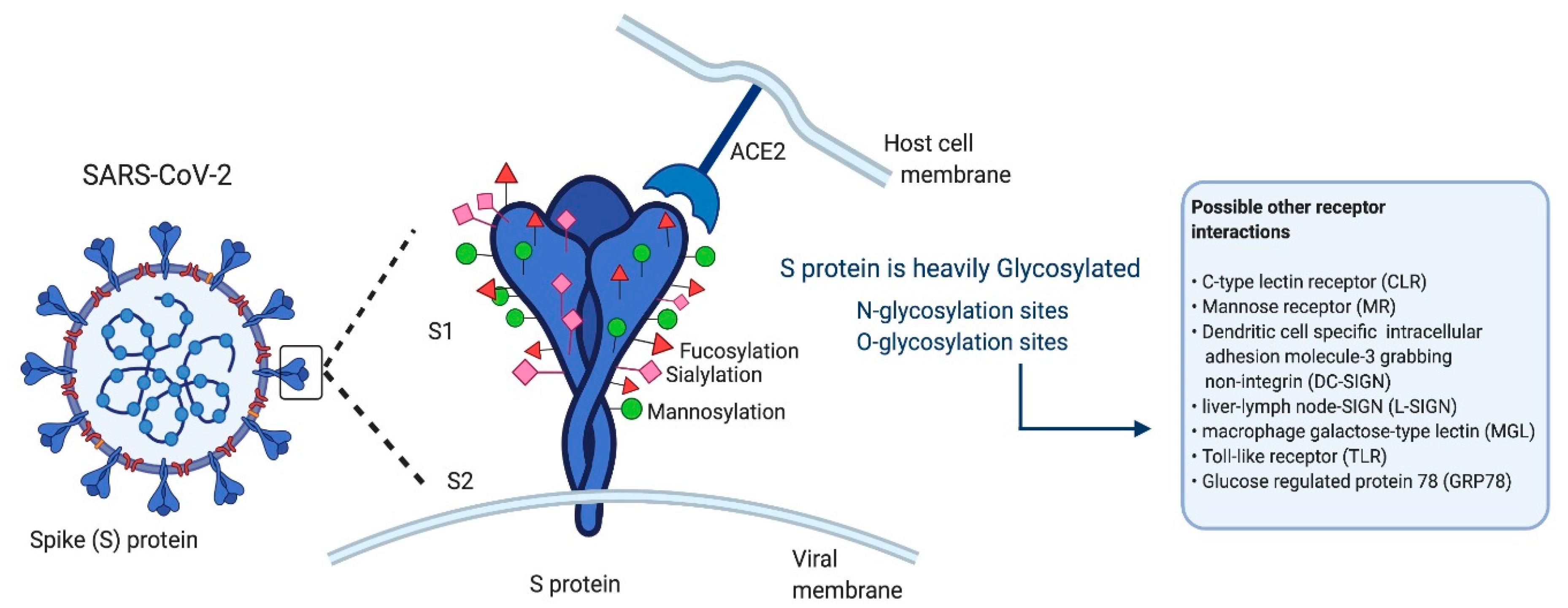This diagram illustrates the structure and interactions of the SARS-CoV-2 virus, focusing on its spike protein (S-protein). Set against a white background, the image starts on the left with a depiction of the virus labeled "SARS-CoV-2 spike S-protein," likely representing COVID-19. The middle section expands on this, showing a detailed view of the S-protein, highlighting its components and modifications such as glycosylation. The S-protein is depicted as a blue, twisting structure adorned with various symbols—green circles, red triangles, and pink squares—indicating specific sites of sialylation, mannosylation, and other types of chemical modifications. The right side of the diagram transitions to the host cell membrane, indicating the S-protein's heavy glycosylation and potential interactions with multiple receptors, such as the ACE2 membrane, C-type lectin receptor, mannose receptor, and the DC-SIGN receptor. The diagram also includes annotations about possible receptor interactions, presenting a comprehensive map of how the spike protein might attach to host cells.